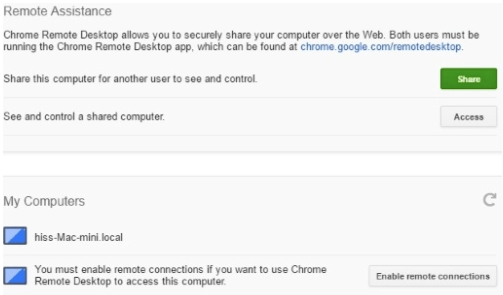A screen capture depicts a section of a website or app interface dedicated to remote assistance. At the top, a prominent gray box features the header "Remote Assistance" and contains a succinct description spread over two lines: "Chrome Remote Desktop allows you to securely share your computer over the web. Both users must be running the Chrome Remote Desktop app, which can be found on the website." Directly below this text, a prompt reads, "Share this computer for another user to see and control," accompanied by a green button labeled "Share" on the right. Further down, another line states, "See and control a shared computer," with a white button labeled "Access" on the right side.

Below this section, there is additional spacing leading to another gray box with the header "My Computers" in a larger font. To the right of this header is a refresh button. Within this box, two lines display icons of blue monitors next to the names of different computers. At the bottom of this section, the message "You must enable remote connections if you want to use Chrome Remote Desktop to access this computer" is visible. To the right of this message is a white button labeled "Enable Remote Connections."